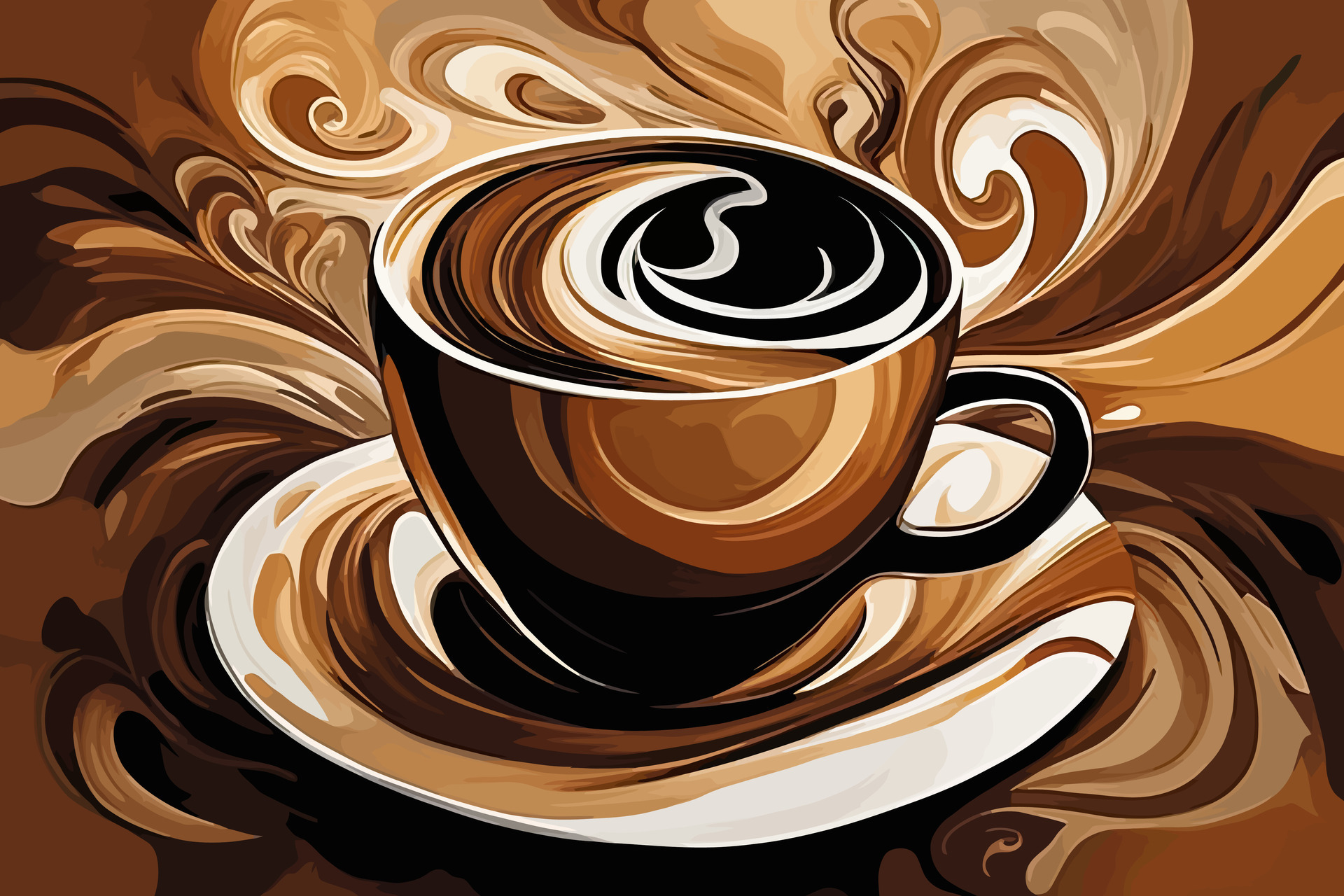This captivating piece of art vividly presents a coffee-themed composition with swirling patterns. Dominated by a rich palette of browns, varying from deep mocha to light cream, the image captures the essence of a freshly brewed cup. At the center is a coffee cup adorned primarily in brown hues with a black handle poised to the right, perched on a saucer that also bears the distinctive swirling motifs. These swirls, in shades of brown, tan, and white, create a dynamic motion across the canvas, reminiscent of the mesmerizing dance of cream as it melds into coffee. The coffee within the cup is a dark brown, suggesting a blend enriched with cream, exhibiting an entrancing swirl. The entire backdrop of the image is alive with these swirls, extending from the bottom to the top, evoking a sense of rising steam and melding seamlessly with the theme.